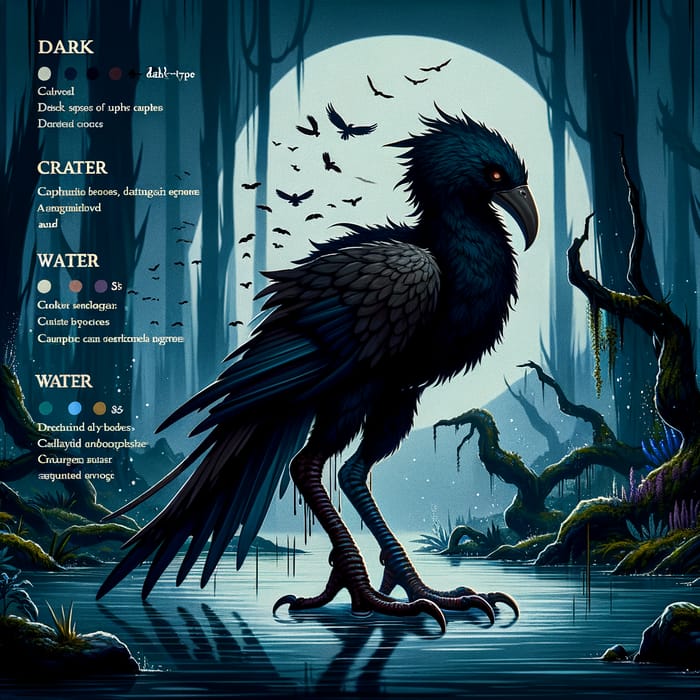This AI-generated digital artwork depicts a large, mystical bird standing atop a body of water in a swampy setting. The bird, which has a phoenix-like appearance, features long legs, sharp claws, and a menacing, glowing yellow-red eye set in a black ring. Its feathers are predominantly dark blue and black, with portions around the head appearing bluish-black and the neck and wing tops displaying shades of gray. The long tail feathers are grayish on the left and bluish-black underneath. This foreboding figure contrasts starkly with its environment: a moonlit forest at night, devoid of leaves and draped in green moss. Silhouetted birds fly against the large, glowing moon, adding to the eerie atmosphere. On the left side, there's text with color palettes beneath headings—dark, crater, water—likely indicative of a video game setting, though the text itself is not in English. The scene combines elements of a surreal, almost mystical experience with high contrast and vivid detail.